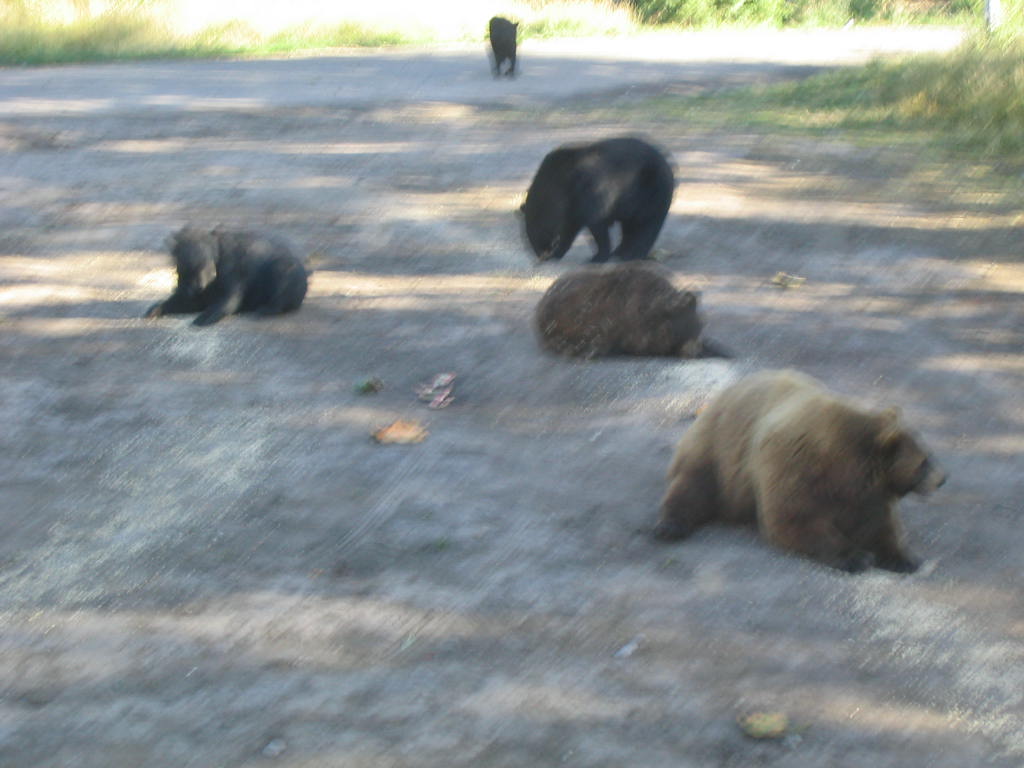Amidst a shadowy trail intersected by a paved road, a very blurry photograph reveals five baby bears in a central open patch of dirt, fringed by peripheral green grass. Illuminated by the dappled sunlight escaping through the tree leaves, the scene captures two brown bears on the right and three black bears on the left. Four of these bears cluster together, with two of the brown bears standing on their feet, seemingly alert and searching for something. The three black bears include two seated on the ground and the third laying down, slightly angled toward its companions. A fifth bear, positioned farther away on the paved road, is either approaching or retreating from the viewer. The image's indistinct quality adds an enigmatic texture, making it difficult to determine the finer details but contributing to its mysterious atmosphere.